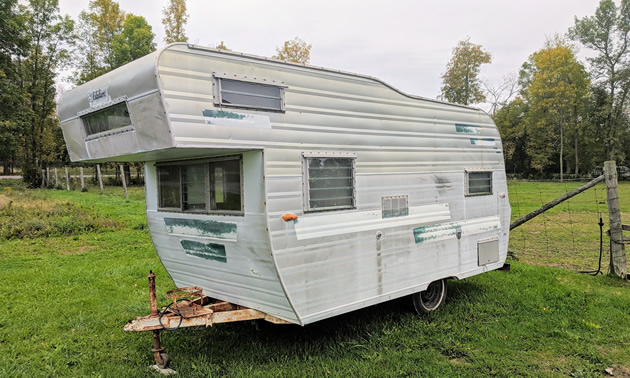The photo features an older style RV camper parked in a green, grassy field. The camper, which appears unused, has a weathered and rustic appearance with off-white metallic siding and patches of green peeling paint, suggesting its age. Rust is visible on the hitch at the front, designed to attach to a vehicle for towing. The structure of the camper includes an overhanging top section, likely serving as a sleeping area, and a total of five windows that can be seen. The camper sits in front of a wooden and wire fence, with an open field extending behind it and tall trees populating the distant background. To the right of the camper, there is a small garden patch, adding a touch of greenery to the scene. The aging and chipped paint contribute to the overall nostalgic aesthetic of the setting.